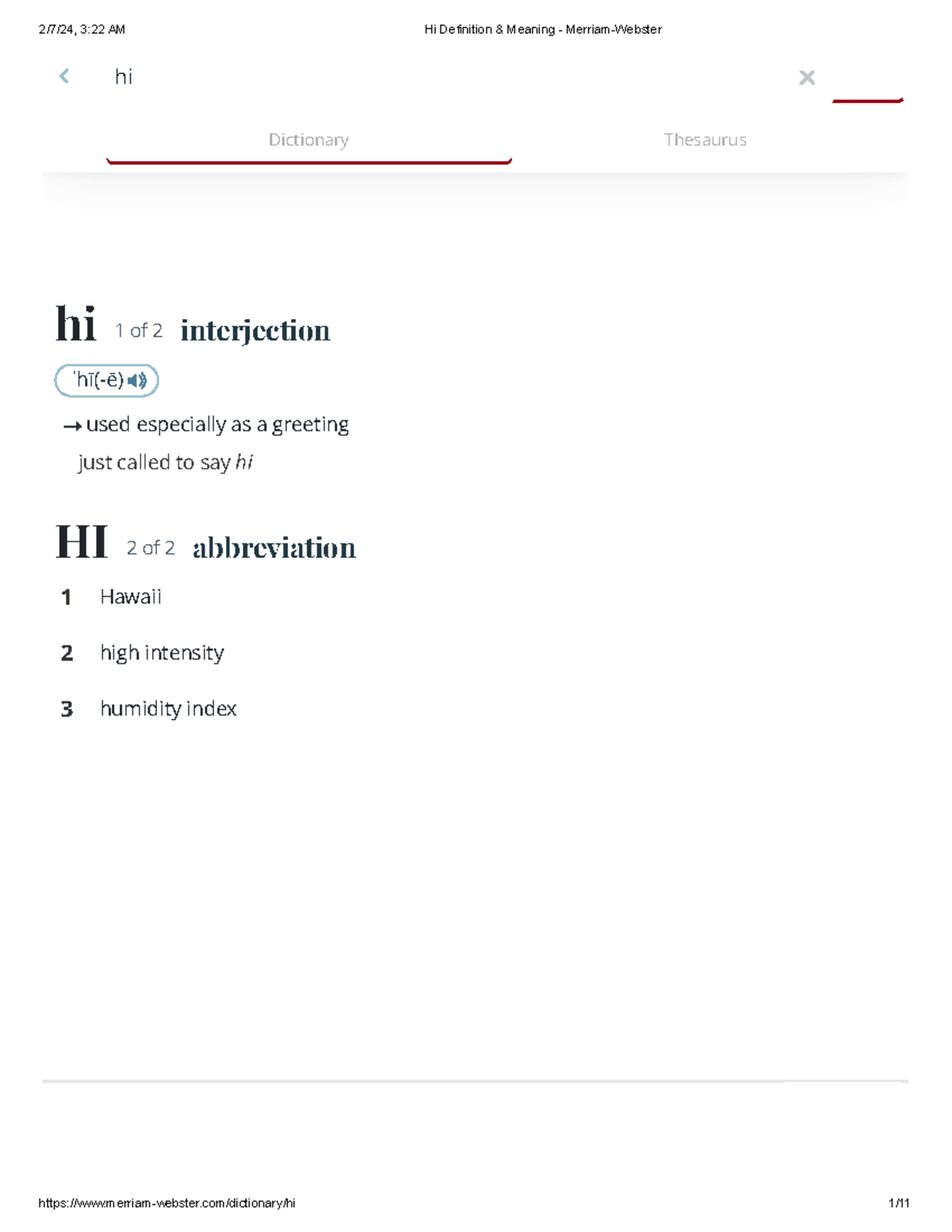This image is a screenshot of the Merriam-Webster dictionary website, taken on a tablet device, as indicated by its wider-than-phone display. In the upper-left corner, the date and time are shown as “2-7-24 3:22 AM.”

At the top-center of the screen, the page title reads: "hi Definition & Meaning - Merriam-Webster." Below this, within the search bar, the word "hi" has been typed, with an 'X' icon available to clear the search input if desired.

Under the search bar, there are two selectable tabs labeled "Dictionary" and "Thesaurus." The "Dictionary" tab is selected, highlighted by a burgundy underline with elegantly curved corners at either end.

The main content area displays two entries for "hi":

1. The first entry is "hi" (one of two), noted as an interjection. The pronunciation is indicated phonetically with special symbols and an accompanying speech icon, which allows users to hear the pronunciation. The definition provided is "used especially as a greeting," exemplified with the italicized sentence "just called to say hi."

2. The second entry is "HI" (two of two), an abbreviation with the meanings listed as "Hawaii," "high intensity," and "humidity index."

The bottom part of the webpage features substantial white space, followed by a thin gray line. At the very bottom right, a text reads "1-11," potentially denoting the page number or a reference metric. The URL of the dictionary page "hi" appears at the lower right corner: "https://www.merriam-webster.com/dictionary/hi".